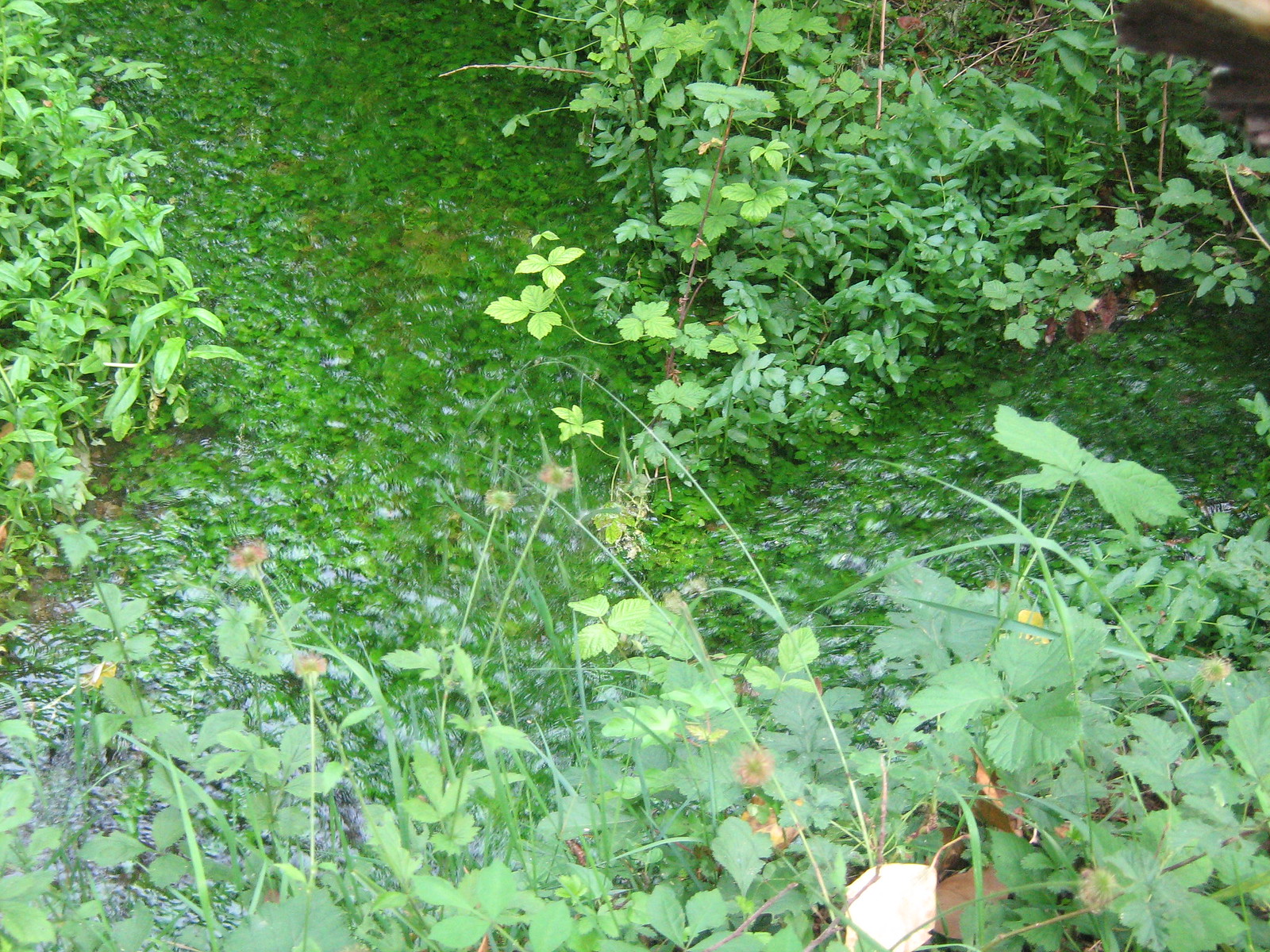In this lush outdoor scene, dense greenery dominates the landscape, creating an overwhelming impression of verdant abundance. The upper half of the image features dense shrubs with varying shades of green leaves, interspersed with thin, twig-like stems. These shrubs frame the scene from the upper left and right corners, enhancing the rich foliage composition. The ground, carpeted with a sea of small, dark green leaves, creates the illusion of a mossy, leaf-strewn walkway stretching from the left side to the center and beyond to the right.

The lower half of the image appears lighter, almost white, as if illuminated by sunlight. This lighter area is somewhat hazy, dotted with lighter green leaves and displaying patches of tall grass blades reaching upwards. Additionally, small, delicate purple flowers can be seen emerging from the bottom left corner, their subtle hues adding a touch of color diversity to the predominantly green palette. 

Hints of brown from twigs and stems peeking through the foliage suggest a natural, unmanicured environment, possibly a swampy terrain, given the rippling water-like effect observed towards the middle and bottom left of the picture. This combination of greenery, light, and water creates a rich, dynamic natural habitat teeming with vegetation.